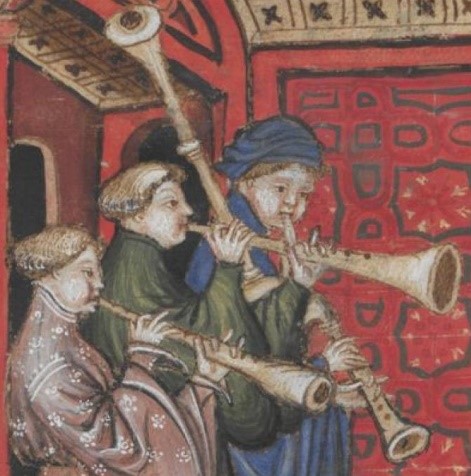This is an image of a painting that appears to have an early Renaissance style, possibly resembling a tapestry or art piece from a textbook. The scene features three men, each playing a unique instrument that looks like a blend between a trombone and a clarinet, possibly identified by Google as linked to the Bagpipe Society. Each figure is depicted in a right profile.

The man on the left wears a pinkish-brown robe adorned with white flowers. The middle figure dons a flowing green shirt, while the individual on the right is dressed in a blue robe and a matching blue hat. Their instruments are tan or beige-colored, long, and stylized to look somewhat like clarinets. The men's faces are characterized by short haircuts and puffed cheeks, giving the impression of active playing.

The backdrop of the painting is a rich red hue with abstract black shapes, evoking an indoor temple setting. The style is loosely impressionistic but also reminiscent of artists like Marc Chagall, with less realistic, more stylized figures and elements. The overall atmosphere of the image suggests it's an old, historically significant artwork portraying musicians in a decorative and symbolic manner.